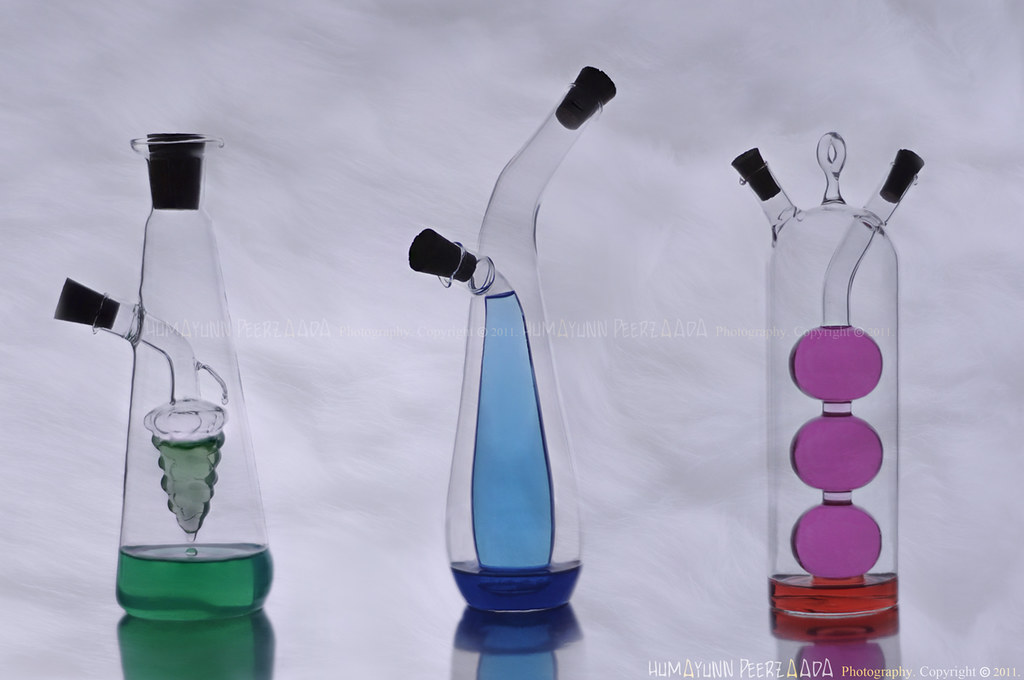This horizontal rectangular photograph features three distinct clear glass beakers, each varying in shape and complexity, set against a slightly crumpled paper-like white backdrop with grey swirls, imparting an almost cloud-like texture. Each beaker, designed as you would see in a laboratory, is intricately detailed with various spouts and all are fitted with black rubber stoppers. 

The beaker on the left has a somewhat triangular shape with a corked top and a side spout, containing a honeycomb or pine cone-shaped inner glass structure holding dark green liquid. The beaker in the middle has a neck that angles upward to the right and includes two spouts; it houses a teardrop-shaped inner bottle filled with dark blue liquid and a larger surrounding liquid of purple. The rightmost beaker, flask-shaped, contains an internal structure of three spherical globes, each connected as part of an elaborate tubular system, and holds a hot pink liquid. The intricate composition and vivid colors hint at both scientific utility and artistic expression.